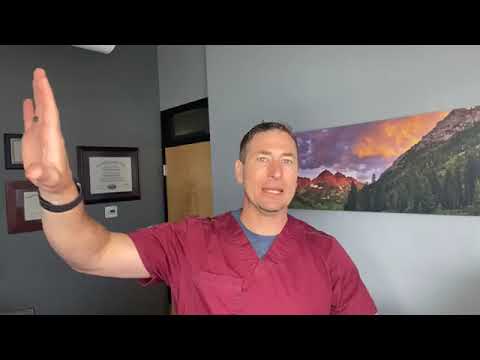In the image, a Caucasian man with very short hair and light-colored eyes stands in the center of a gray-walled room, which appears to be an office. He is dressed in a red V-neck medical uniform with short sleeves over a gray t-shirt and has a wristwatch on his right hand. His right arm is raised, palm facing up, and his mouth is slightly open, as if he is explaining something.

To the left of the man, three framed certificates or diplomas are displayed on the wall, featuring black, reddish, and tan frames. In the background on the left side, a brown wooden door leads to a hallway, while on the right side, a long rectangular landscape painting depicting a fiery sky, red mountains, and some grass hangs on the wall. The image has thin black borders at the top and bottom, framing the scene.